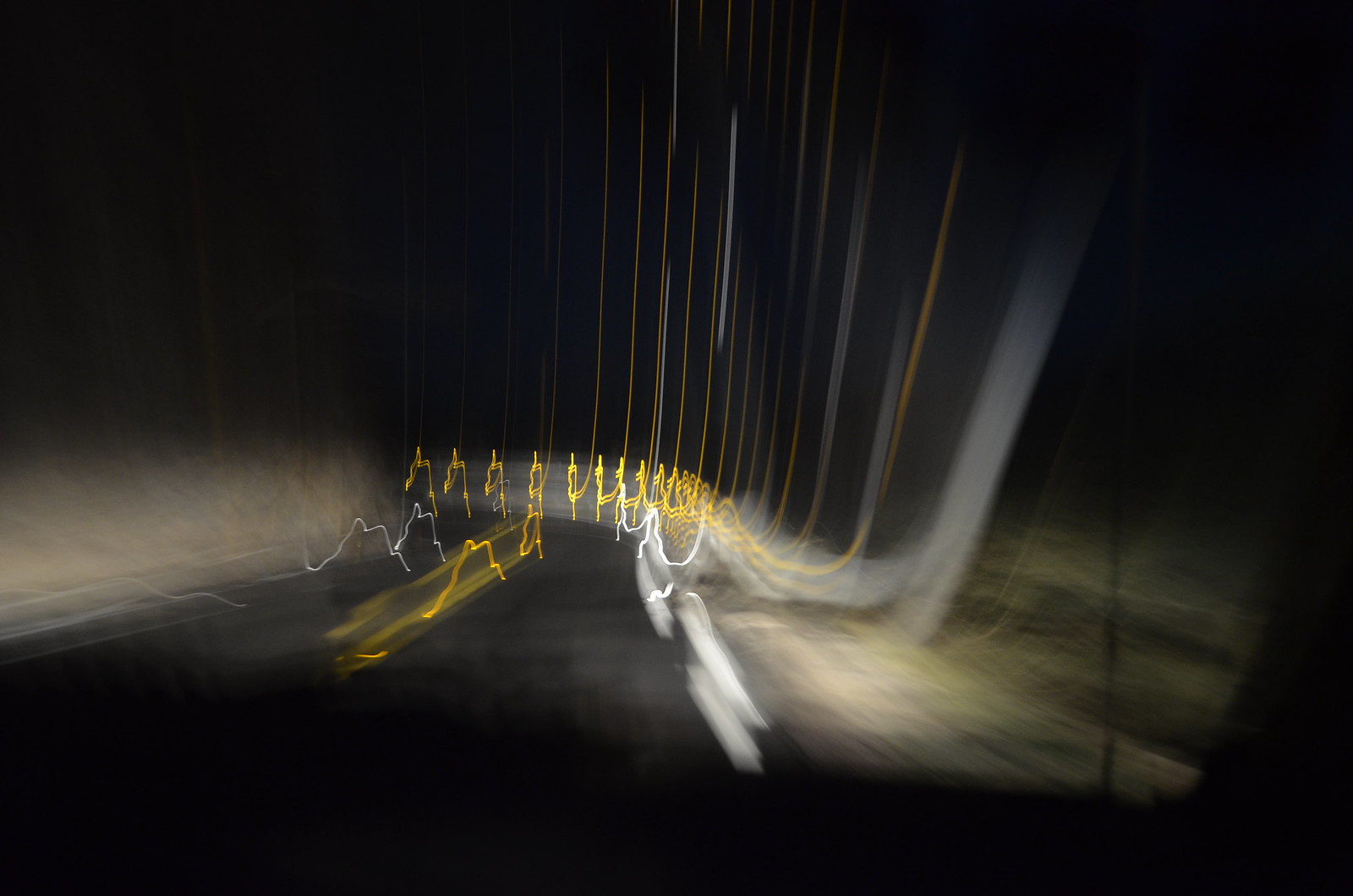The image features an abstract composition with a blurred effect that obscures precise details. Dominating the scene are yellow and white lines that stretch across the picture. In the middle, these lines morph into squiggles before shooting straight upwards into more rigid, straight formations. Interspersed among the yellow and white lines are slightly wider gray lines, adding a contrasting element to the color palette. The ground is a solid black with two blurred yellow lines running across it, enhancing the abstract nature of the artwork. A light source emanates from behind the image, adding a glow that subtly illuminates the scene, while the background remains entirely black, creating a stark contrast that highlights the vibrant lines in the foreground.